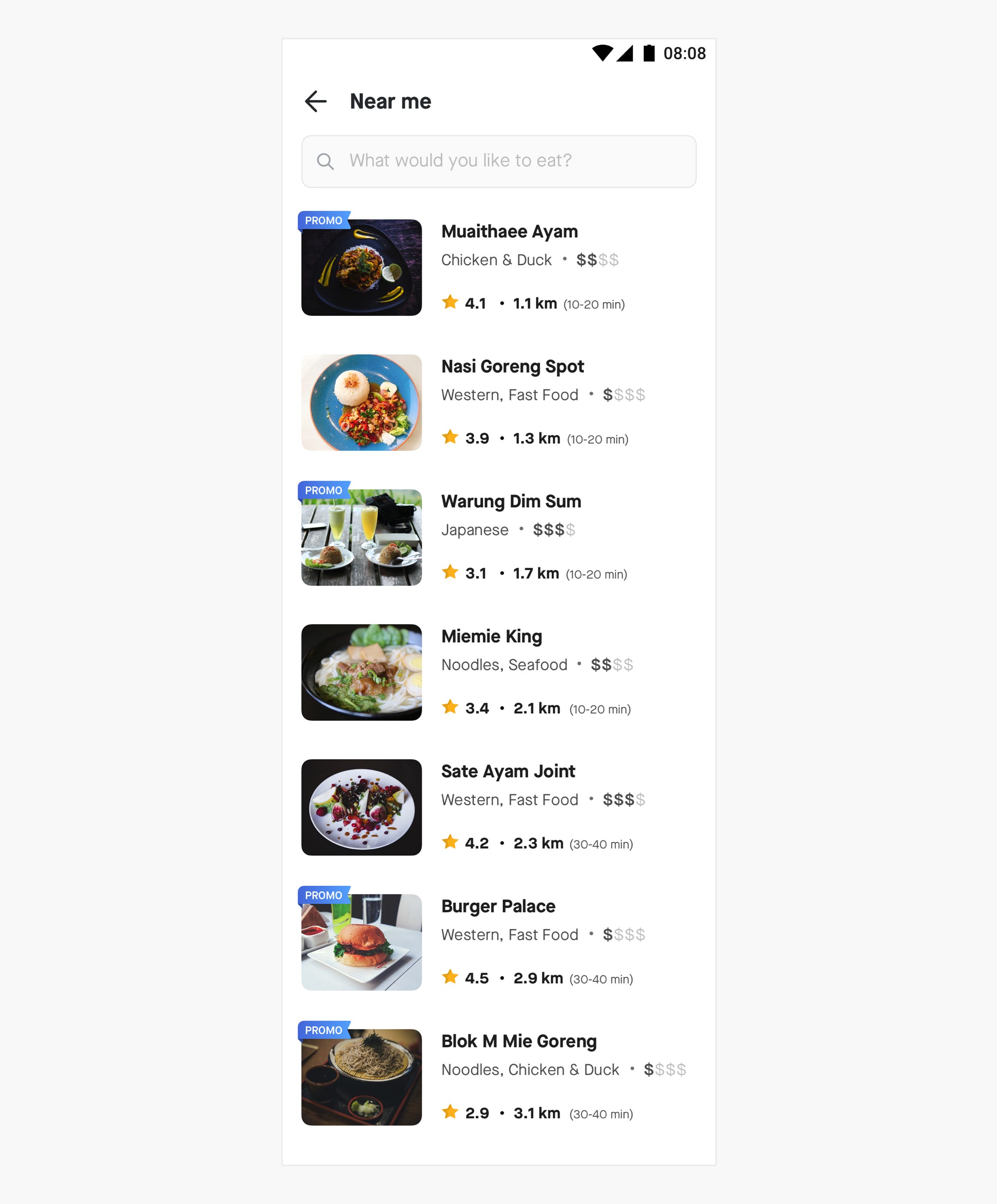Screenshot of a smartphone at 8:08 AM displaying a list of seven restaurants in a foreign language. Each entry includes a photo selected by the restaurant, the restaurant’s name, the cuisine type, an expense indicator symbol, a star rating, and the distance from the current location. The top restaurant is "Mayutai Ayam" and the bottom one is "Bok Em Mi Goreng."